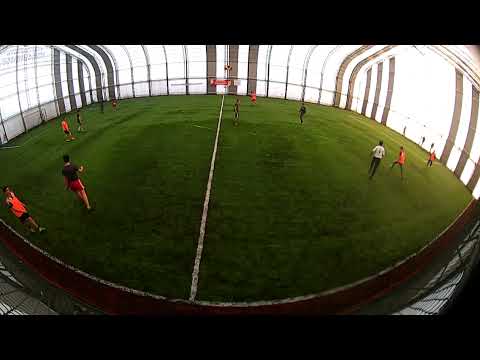This is a panoramic photograph with a fisheye distortion, capturing an indoor soccer match. The lush green turf appears somewhat circular due to the camera lens, though it's normally rectangular. A prominent white line runs down the middle of the field. The walls surrounding the turf are bright white and translucent, likely allowing natural light to stream through. The view does not include the ceiling, adding to the spacious feel of the facility. Soccer players wearing either pink (or possibly orange) tops paired with black shorts, or vice versa, are scattered across the field. A referee in a white shirt and black pants is also visible. Goalposts are present at either end, and in the background, there appears to be either a banner or a scoreboard.